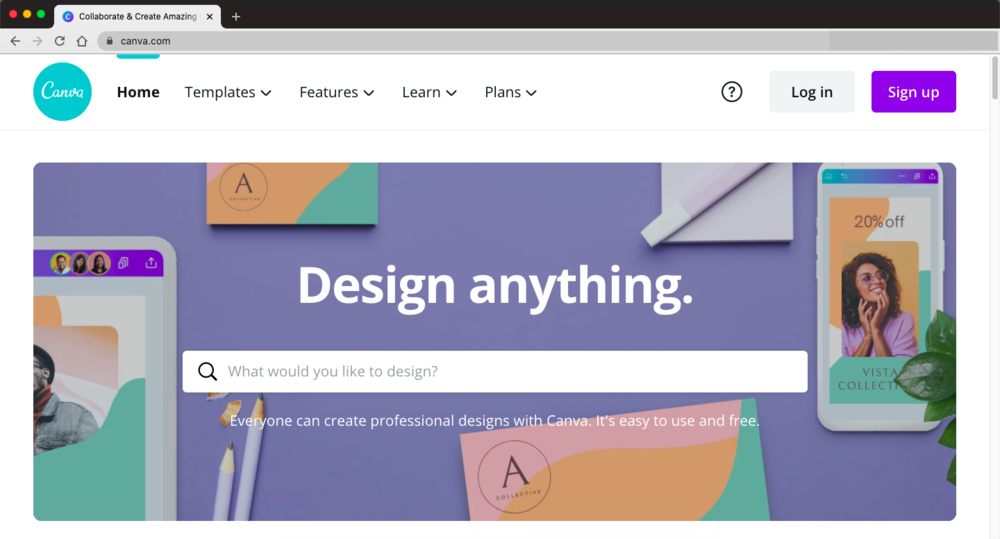**Detailed Image Caption:**

The image is a screenshot of the Canva website viewed within a web browser. At the topmost part of the image is the browser user interface. On the top left corner, three circular buttons are visible—red, yellow, and green—set against a black background, indicating typical browser window controls. To the right of these buttons, the browser tab is shown, featuring the blue Canva logo icon. The tab's text reads, "Collaborate and Create Amazing," followed by an 'X' for closing the tab.

Next, we see the browser's address bar, containing the URL "canva.com," accompanied by a padlock icon symbolizing a secure connection. To the left of the URL field, there are icons for 'home,' 'reload,' and navigation buttons for 'back' and 'forward'.

Below the browser's UI, the webpage content begins. At the top left of the Canva website header, the white cursive Canva logo is displayed inside a blue circular icon. Adjacent to this are the main navigation links: "Home," "Templates," "Features," "Learn," and "Plans," each with dropdown menus. "Home" is bold and black, underscored by a distinctive blue line above it, signifying the active page.

To the further right of the navigation menu, a question mark icon encircled is present, alongside a gray background 'Log in' button and a lavender or purple 'Sign up' button.

Below the navigation bar is a thin gray demarcation line. The white background continues, hosting the main hero section. This section features a prominent rectangular image with text overlaying it. The text reads, "Design anything" in bold white letters. Beneath this, a search bar is displayed, prompting with the text, "What would you like to design?" and displaying a search icon to its left. Additional subtext below the search bar explains, "Everyone can create professional designs with Canva. It's easy to use and free."

The hero image backdrop appears to be a wall adorned with sticky notes or images resembling phone screens. This screenshot captures the essence of Canva's user-friendly interface and design capabilities, neatly structured under a seamlessly integrated browser window.